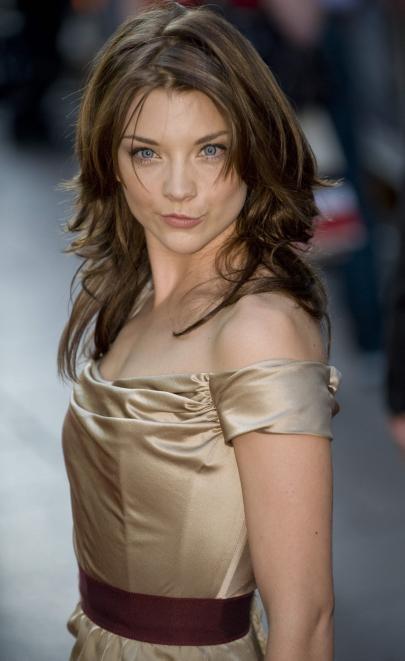This photograph captures a woman who closely resembles a young Kirstie Alley or could be an actress from Game of Thrones. She stands posing sideways while looking forward, her lips pursed in a playful, duck face expression. Her shoulder-length, brown hair features a zigzag part and cascades into curls and waves at the bottom. She wears a fancy evening gown made of shimmering, silky material in a gold-tan hue. The dress is sleeveless with partial sleeves around her shoulders and is complemented by a burgundy or reddish-brown sash around her waist. The background is predominantly blurred and features indistinct hues of white, red, and dark gray, ensuring the focus remains on the model with her striking blue eyes. The picture is in a vertical, rectangular format.